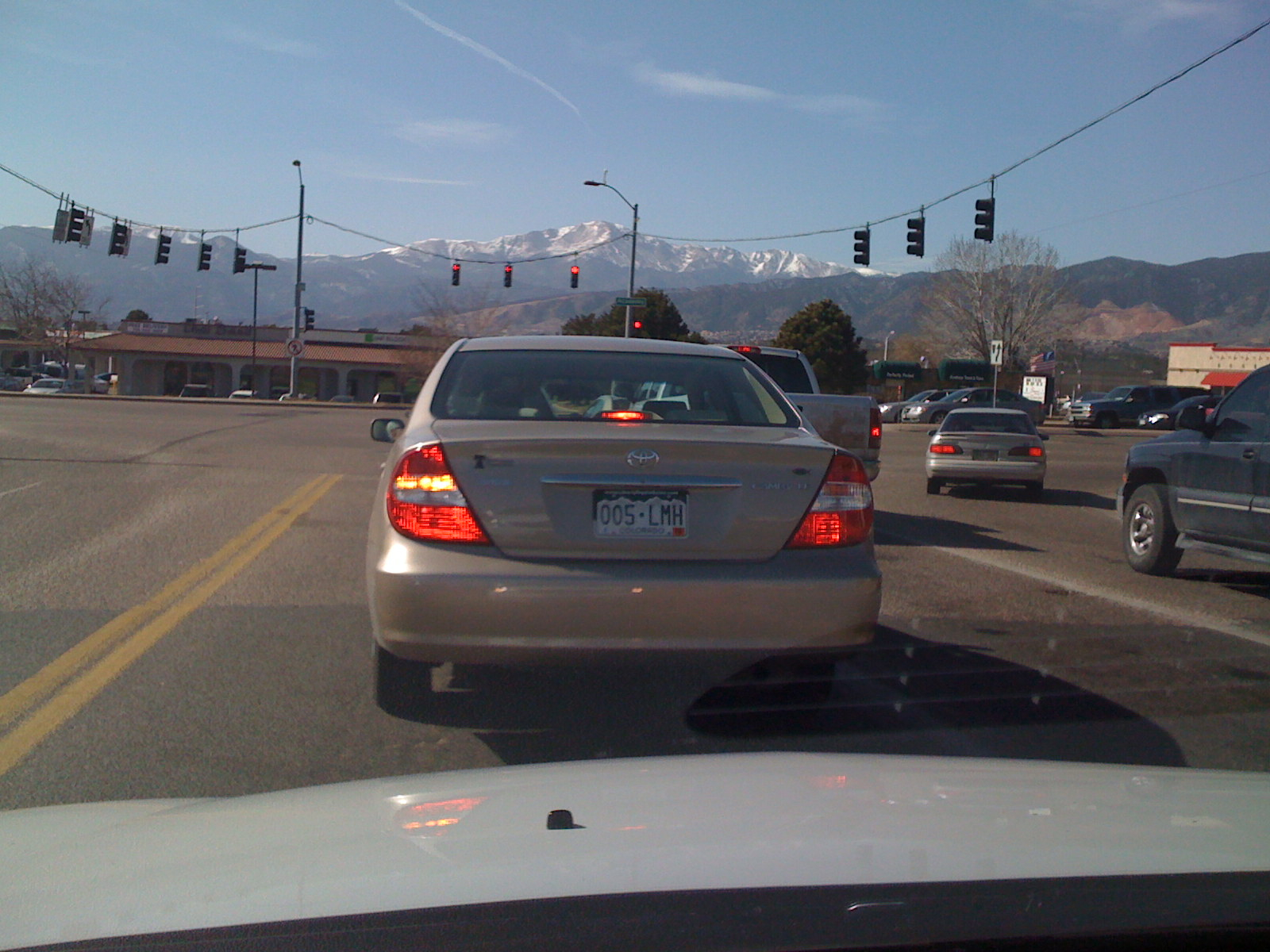This color snapshot captures the scene from inside a car, potentially from the passenger side, looking through the windshield towards a bustling intersection in what appears to be Colorado. The hood of the vehicle we are in is visible, displaying a white color with some reflections off the windshield. Directly ahead, a light-colored Toyota sedan with Colorado license plate 005LMH has its brake lights on, stopped at a red light. To the left of the Toyota, a dark-colored pickup truck and another sedan, likely a Ford Taurus, are also waiting at the intersection, their brake lights glowing. To the right, a black pickup truck and another vehicle are positioned, with the scene framed by double yellow lines on one side and a white line on the other.

The intersection is well-defined with three strands of traffic lights hanging from wires, as well as additional streetlights scattered around. On the far side of the crossroads, there’s a long, low building that might be a bank, and a wider shopping area can be seen to the left beyond the intersection. The setting reveals more buildings stretching off to the right, giving a sense of a busy, urban environment.

In the far background, majestic snow-capped mountains rise prominently, with smaller, greener mountains in the foreground, adding to the scenic beauty. These natural features dominate the horizon beneath a light blue sky with sparse clouds, framing the scene inside the car with a picturesque Colorado backdrop.